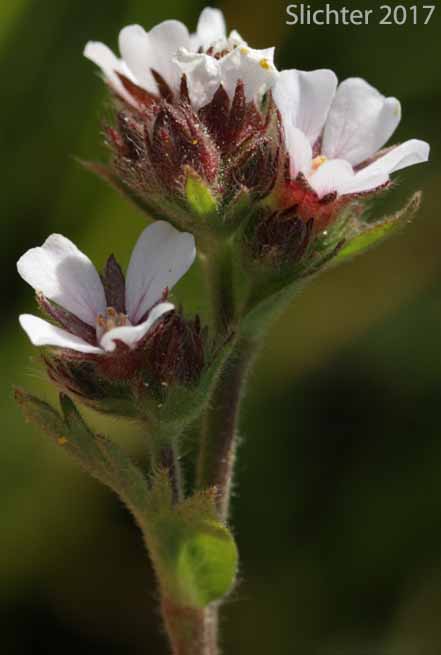This image, either a photograph or a hyper-realistic piece of art, titled or credited as "Slichter 2017," captures a stunning close-up of a unique flower against a blurred backdrop of dark and light greens. The portrait-mode composition centers on a green, fuzzy stem sprouting into multiple sections, each adorned with intricate white flowers emerging from vivid red buds. The flowers feature delicate, shadowed white petals, with some showing hints of yellow. Surrounding each bloom are green leaves, some with shades of red. Notably, there are several unopened buds poised to reveal their beauty, adding an element of anticipation to the scene. The fine texture of the stem, buds, and petals is meticulously captured, showcasing the flower's intricate beauty in remarkable detail.